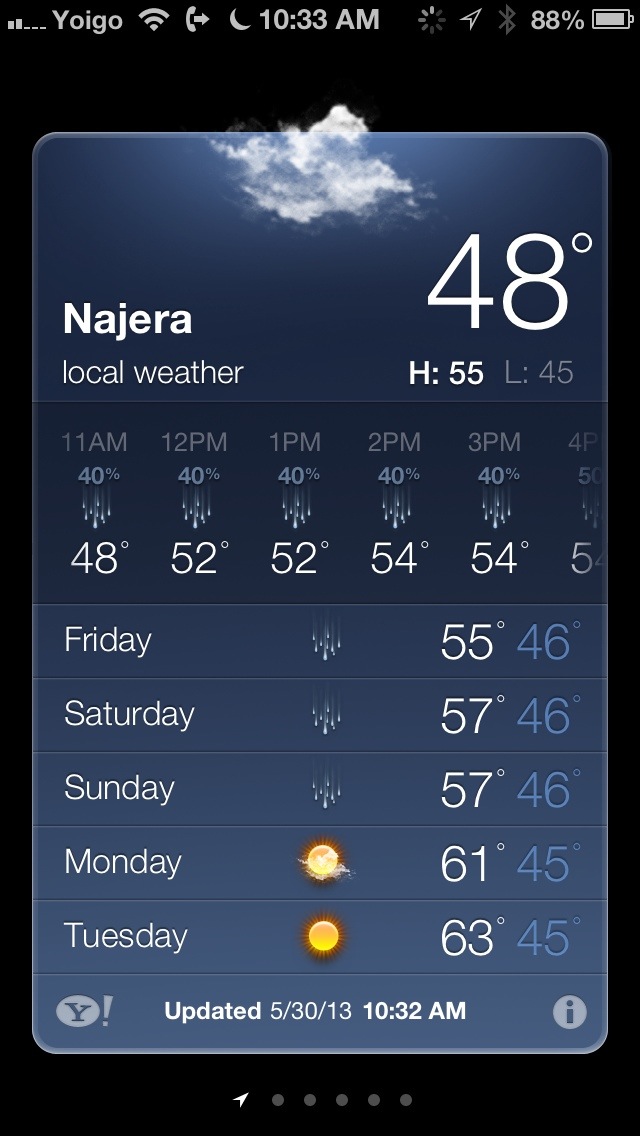A smartphone display screen is captured in this detailed image. The screen shows various icons: signal bars indicating cellular strength, the text 'YOIGO', Wi-Fi signal bars, a phone icon with a right arrow, and a crescent moon symbolizing Do Not Disturb mode, all displayed at the top. The device time is noted as 10:33 A.M., and the battery is charged to 88%, with Bluetooth enabled. The predominantly black screen features a prominent blue vertical rectangle in the center with a cloud graphic and weather information for Nigeria. The weather details are as follows: current temperature is 48°F, with a high of 55°F and a low of 45°F. Hourly forecasts are listed: 11 A.M. shows 48°F with 40% chance of rain, 12 P.M. and 1 P.M. both at 52°F with 40% chance of rain, and from 2 P.M. to 3 P.M. 54°F with 40% chance of rain. The forecast summary includes Friday through Tuesday, noting frequent rain followed by partly cloudy and sunny days. The YouTube logo appears at the bottom of the screen, with an update time-stamped at 10:32 A.M. on May 30, 2013.